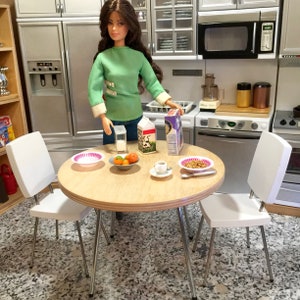In the image, a doll with long, sleek black hair cascading halfway down her back is depicted in a detailed and vibrant play kitchen setting. The doll is dressed in a charming green sweatshirt with slightly rolled-back black sleeves, revealing white cuffs. 

The background showcases a variety of play kitchen appliances designed to emulate stainless steel, including a refrigerator, an over-the-range microwave, an oven, a stovetop, and a dishwasher. A sink with a dish strainer sits just behind the doll, adding to the kitchen's realism.

In the foreground, the doll stands in front of a round wooden table set with two white chairs. She is placing one hand on a box of cereal while her other hand rests on another indistinct box due to the image's focus. The table is adorned with an empty bowl to the left, a central bowl filled with a colorful assortment of fruit, and another bowl on the right containing a brownish substance with a spoon lying next to it. The scene captures a lively moment in this meticulously arranged miniature kitchen.